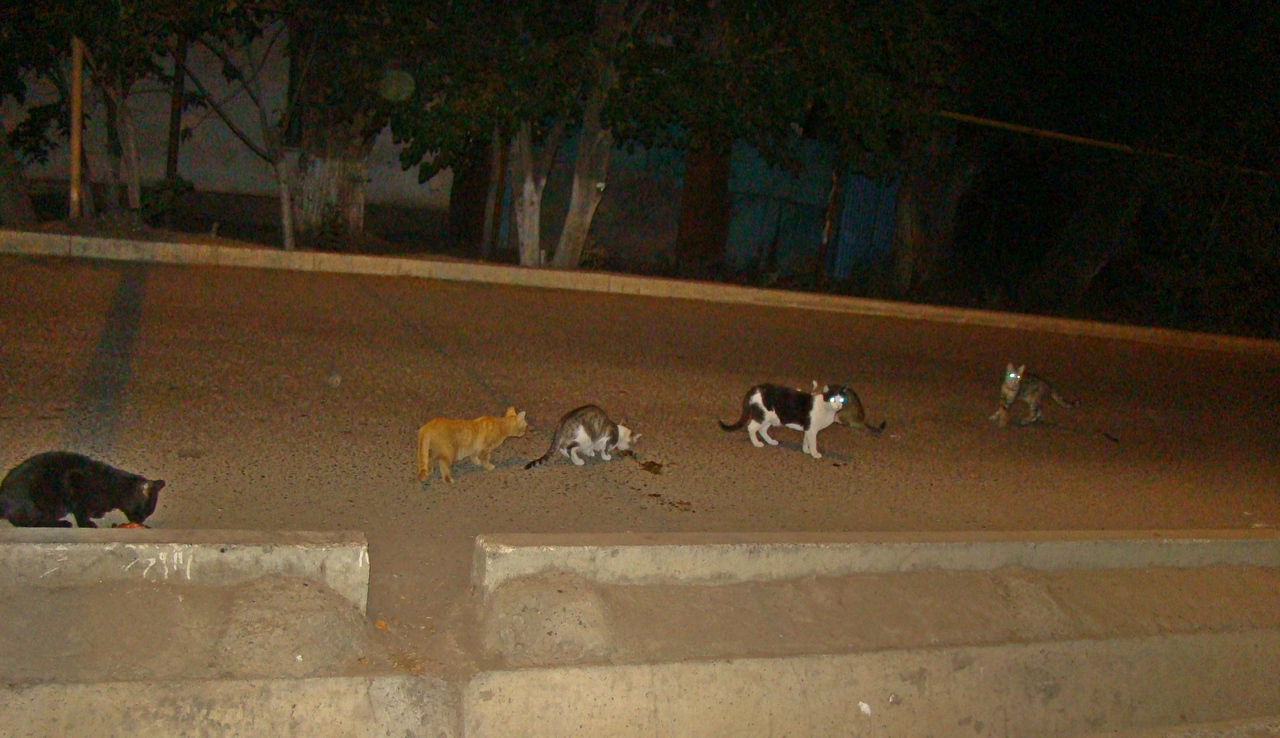This nighttime exterior shot captures six cats gathered on a dark, gray concrete road, punctuated with a high curb that resembles a freestanding divider. The scene is illuminated by an unseen light source, possibly the camera flash, causing two of the cats' eyes to glow prominently. The background features the silhouette of trees with sparse leaves and a bluish single-story building. The cats, spread out from left to right, appear to be eating or sniffing at something on the road that may be roadkill or some kind of food.

Starting from the left, the first cat is black and is bent down eating. To its right is an orange tabby, followed by a gray and white cat, both of which seem to be engaging with something on the ground. The next is a white cat with black spots, resembling a cow pattern; its eyes reflect the camera's flash. Behind this black and white cat is a small, partially occluded cat whose tail and ears are visible. Farther to the right, a gray tabby cat and another gray cat are positioned, both facing the camera with their eyes shining brightly. The detailed composition of colors includes gray, white, orange, black, and some mixed patterns, creating a spread of feline variety against the muted urban backdrop.